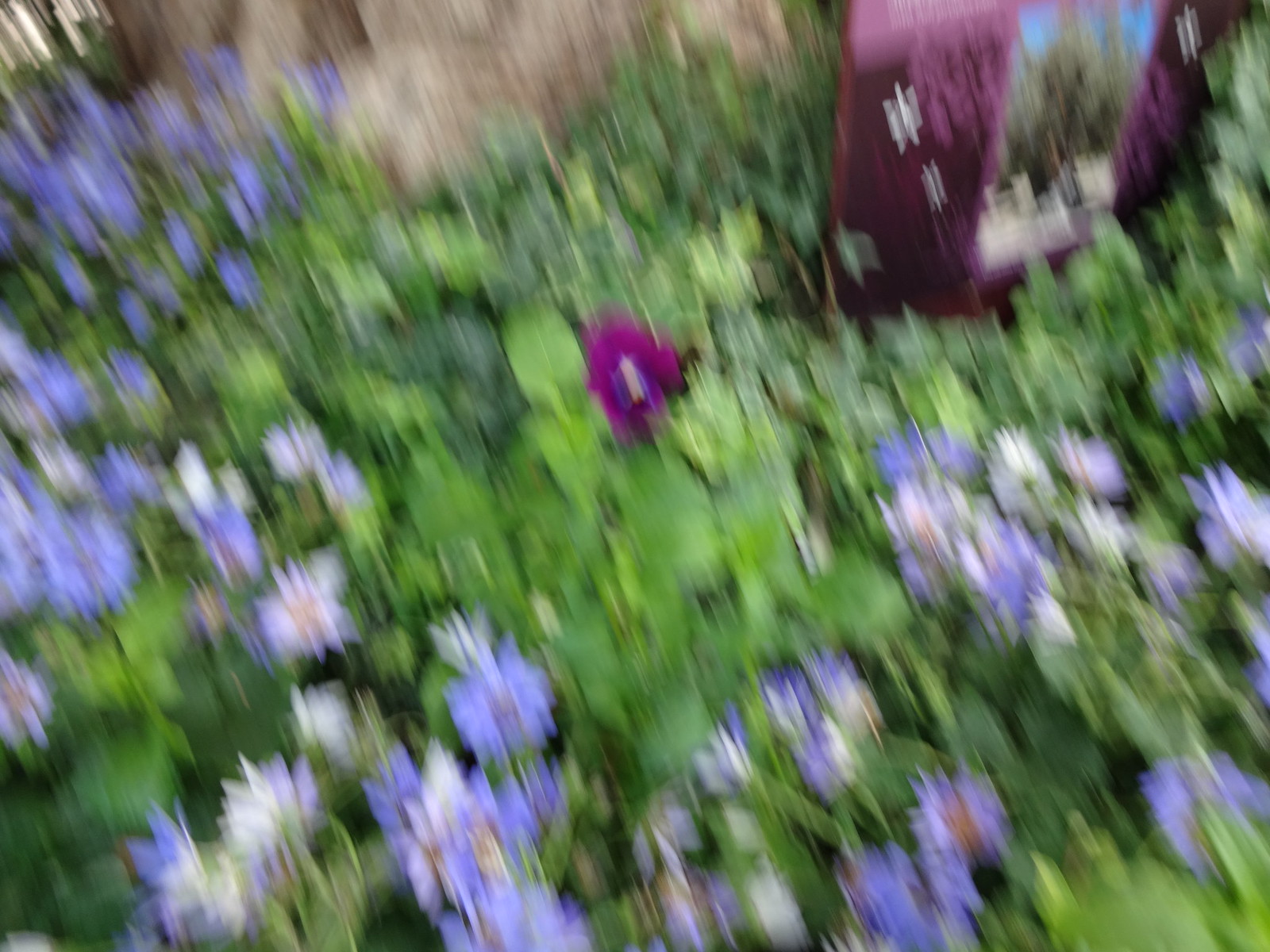This is a very blurry close-up image of a lush garden. The entire picture is dominated by green leaves interspersed with flowers of varying shades, such as light purple, dark purple, light blue, and white with yellow centers. The center of the image showcases a singular dark purple flower that starkly contrasts with the surrounding greenery. In the top left corner, blurry sunlight can be seen shining around what appears to be the base of a tree. The top right features a purple-bordered rectangle or sign, which contains an indistinct photo or image within its center. Additionally, there are more purple flowers scattered throughout the bottom and right side of the picture, forming a triangular pattern up the right edge.